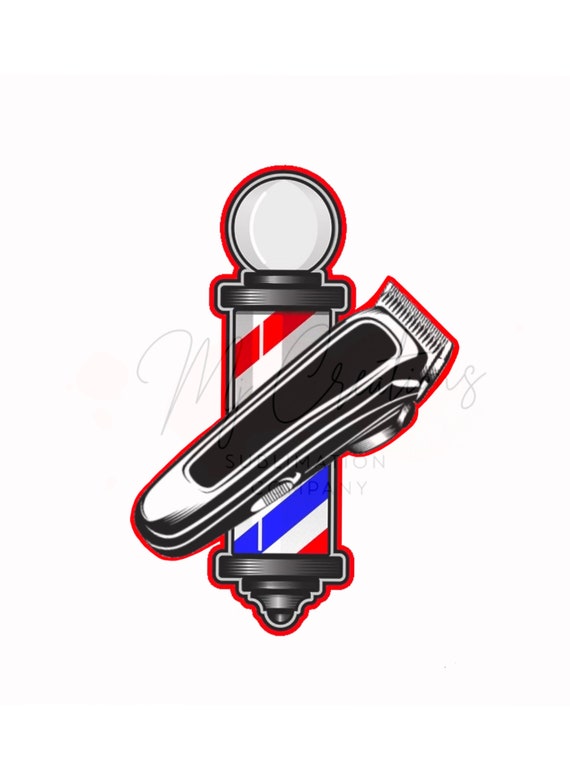This digital art piece showcases a centrally placed cartoon depiction of a classic barbershop pole, featuring its iconic spinning red, white, and blue stripes and topped with a white circular bulb. The pole is outlined in red and stands prominently against a stark white background. In front of the pole and intersecting its red outline, there is an electric razor angled towards the top right of the image. The razor, primarily black, is also accented with a red outline and appears more rectangular with rounded edges, featuring distinctive oscillating metal teeth for trimming hair. Above the entire composition is a semi-transparent handwritten signature that is difficult to decipher, and similarly, a semi-transparent watermark is present below the main elements, adding a subtle branding layer to the scene. The cohesive design elements suggest a possible logo or branding image, capturing the essential tools of a barber's trade.